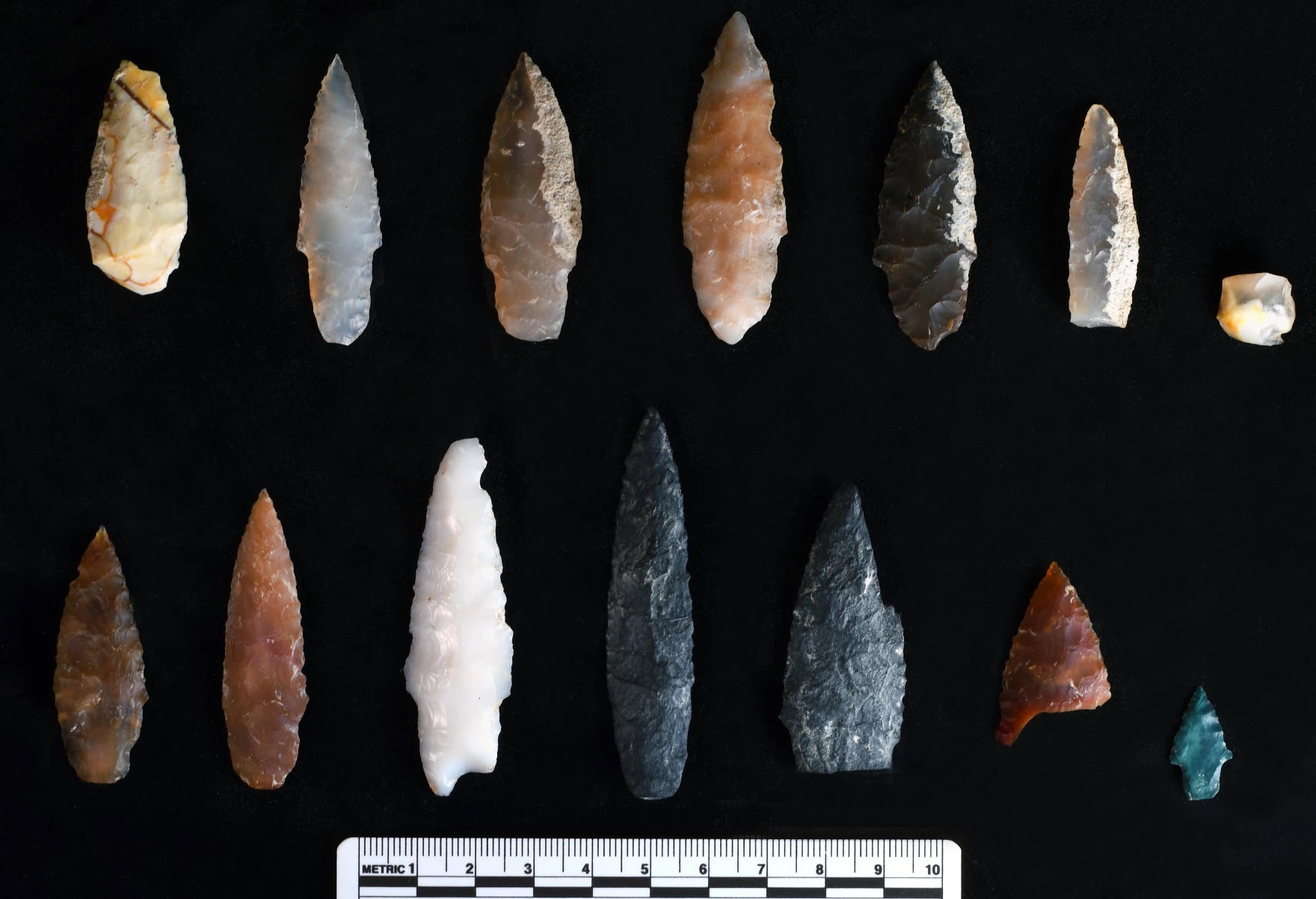This image features 14 meticulously arranged stone artifacts that resemble arrowheads, set against a stark black background. The objects are aligned in two rows of seven at the top and bottom of the frame. At the bottom center lies a white ruler marked in centimeters, with black numbering and hash marks for millimeters and centimeters, featuring a black-and-white rectangular checkered pattern at the edge. The artifacts, varying in color and material, display a range of hues including yellowish-white, silver-white, brownish-white, orangish-white, pure white, brown-black, dark brown, red-orange, and teal. Each piece appears to have a smooth stone texture, sharply tapering to a point at the top, though some show chips on their surfaces. The size and shape of each stone are similar, highlighting their uniform crafting while emphasizing their diverse material composition.